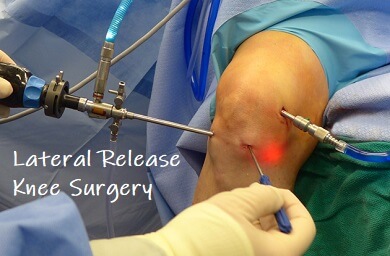The image captures a detailed scene of lateral release knee surgery, specifically noted in white text on the lower left-hand side. At the center of the photo is a patient's knee, positioned and bent over a surgical bed. The focal point showcases a doctor's gloved hands manipulating various surgical instruments. On the right side, the doctor holds what looks like a screwdriver, piercing through the skin. In the left hand, the doctor grips another pointed medical instrument, possibly a drill or saw, also inserted into the knee. Multiple small incisions can be seen where these tools are inserted, rather than large cuts. Additionally, a red laser light illuminates the lower right part of the knee, enhancing visibility for the surgical procedure. This appears to be either a screenshot or frame from an instructional or informational video on knee surgery, underlining the meticulous and technical aspects of the procedure.